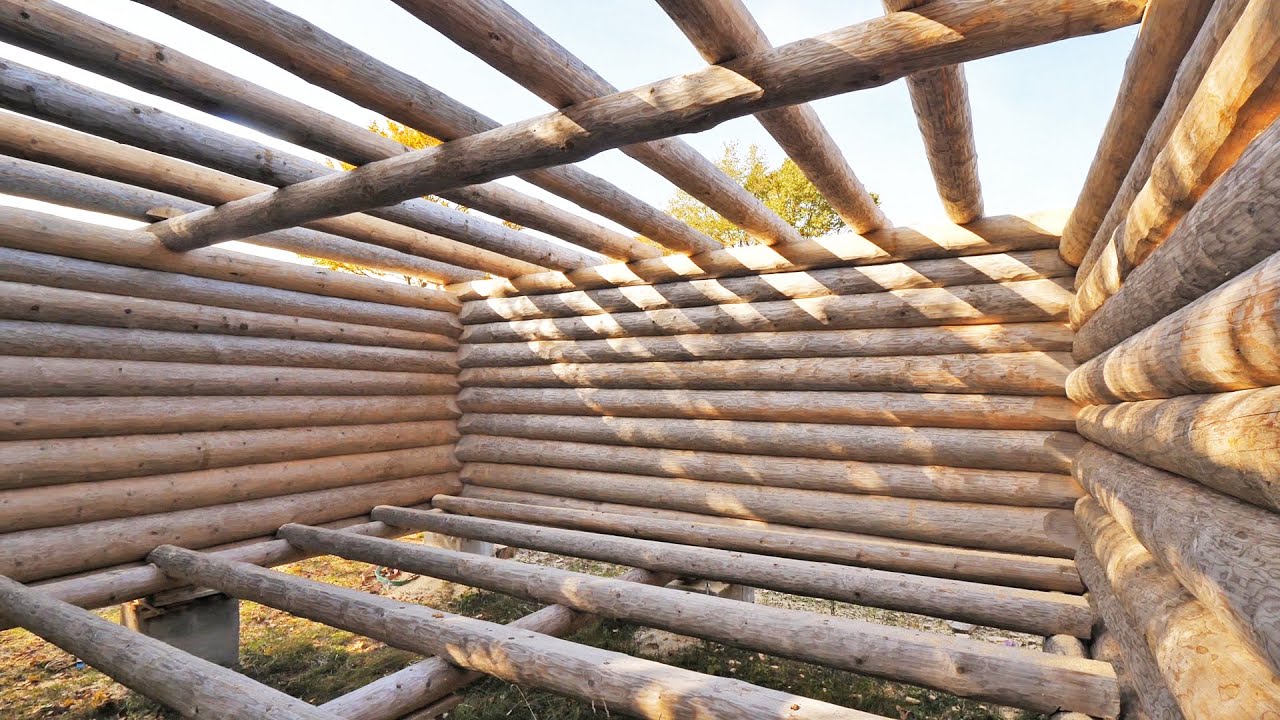The image depicts a wooden structure resembling a log cabin under construction, with defining characteristics of both an open cage and a skeletal frame. Made from thin, de-barked logs, the structure features beams arranged closely together on the left, back, and right sides, creating a solid, unbroken appearance. The floor and ceiling beams are spaced about a foot apart, revealing glimpses of the foundation and allowing sunlight to stream through, casting shadows on the smooth wooden surfaces. Positioned outdoors, the incomplete structure rests on two concrete blocks, with dirt and debris beneath and surrounding foliage visible in the background. A vivid blue sky and trees add to the sense of an open, sunny day, further highlighted by the bright light filtering through the exposed framework.